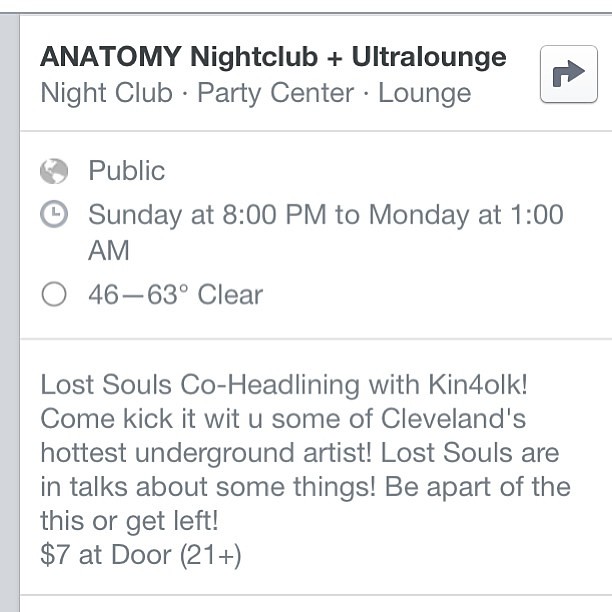The image is a screen capture of a promotional event listing for a nightclub. The background is predominantly gray with a thin gray line running vertically on the left. The event is hosted at Anatomy Nightclub + Ultra Lounge, described as a "Nightclub, Party Center, Lounge." The event is open to the public and scheduled for Sunday at 8 p.m. until Monday at 1 a.m., with the weather forecast indicating clear skies ranging from 46 to 63 degrees. The event features "Lost Souls" co-headlining with "Kinfolk," a name stylized as "KIN4OK." The promotion invites attendees to "come kick it" with some of Cleveland's hottest underground artists, hinting that "Lost Souls" are discussing future projects. The entrance fee is $7 at the door, with an age restriction of 21 and over. Additionally, there's a small globe icon next to the word "Public," and a forward arrow in the top right corner of the image, adding to its sleek design.